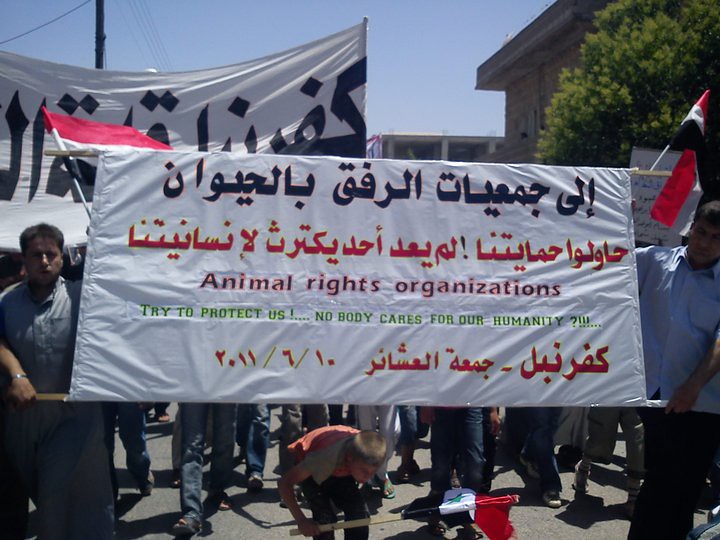This image captures a vibrant protest march taking place on an asphalt road in the middle of the day. Approximately 25 people are seen marching, many holding flags and banners. The central focus is a large white banner with a mix of Arabic and English text. At the top of the banner, Arabic text is written in black and red. Beneath it, in purple English letters, it states "Animal Rights Organizations," followed by "try to protect us, nobody cares for our humanity" in green. More Arabic text in red is found below the English message. 

On the left and right of this central banner, two individuals are seen holding it up; one dressed in a gray shirt and dark pants, the other in a blue shirt and dark pants. Directly beneath the banner, a child in a red shirt and black pants is crouched down, holding a small red, white, and black flag. In the background, another sign with Arabic text, mostly obscured, is visible along with additional red, white, and black flags. 

There are buildings in the distant center and top right part of the image, with a tree beside the rightmost building. The scene is set outdoors under a clear sky, underscoring the daytime setting of the protest. The details and colors—such as light blue, black, white, red, gray, green, purple, pink, and tan—add to the vibrant and dynamic nature of the protest march captured in this image.